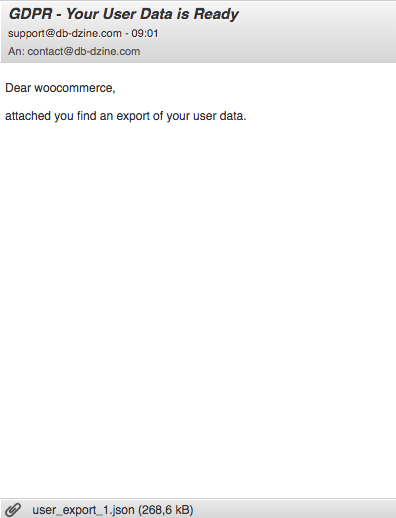In this image, a grey square is situated at the top. On the left side of this square, the text reads "GDPR - Your User Data is Ready" in black font. Below this, in a lighter black font, it states 'support at db.dzine.com - 09-01', followed by 'contact at db.dzine.com'. 

On a line with a white background and black font, it says "Dear WooCommerce". The next line continues with, "Attached you will find an export of your user data." 

Following a large white space, there is another grey square at the bottom. Inside this grey square, there appears to be a greyish image of a paper clip to the left. Next to the paper clip, the text "user-export-1.json" appears in black font, with the file size "268.6kb" enclosed in brackets.